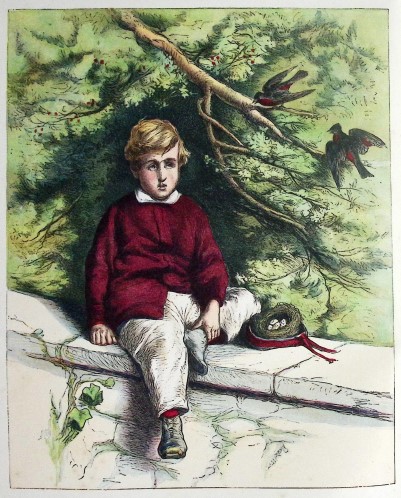This is a detailed illustration, possibly a watercolor painting from an old book, depicting a young boy of about 7 or 8 years old, seemingly from the Edwardian or Victorian era. The boy, who has short, tousled blonde hair and a sad expression, is seated on a gray stone garden wall adorned with ivy. He wears a wine-red cardigan over a white shirt, matching white trousers, black lace-up leather shoes, and red socks. His left leg is tucked in, with his left hand holding onto his ankle, while his right hand rests beside him. Perched on a tree branch above his head on the right are two birds, black and maroon-red in color, seemingly voicing their concern at the boy. This reaction appears to be because he has taken their nest, which is tied with a bow and contains four white-speckled eggs, and placed it on the ledge in front of him. The scene is lush with foliage from the boy's torso up, creating an intricate backdrop behind the birds and the branch.